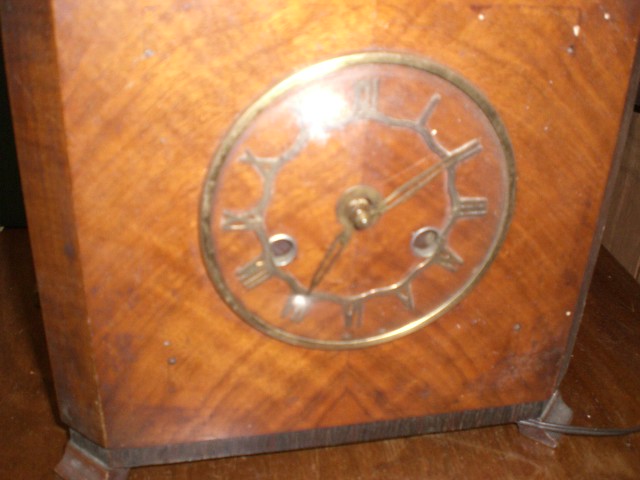A highly decorative table clock crafted from wood takes center stage in this image. The clock features a sophisticated wood block design adorned with brass inlays. The brass constitutes not only the numbers but also the hands of the clock and an embedded frame around the timepiece. The wood exhibits a unique texture, resembling a herringbone pattern, although it is distinctly wood grain. The grain is artfully cut into two pieces, which meet to form a pyramid-like pattern, enhancing the clock's aesthetic appeal. The clock rests on a table, supported by small metal feet, and a visible cord extends from it. The photograph appears to have been taken with a flash, as evidenced by the bright light illuminating the top of the image.